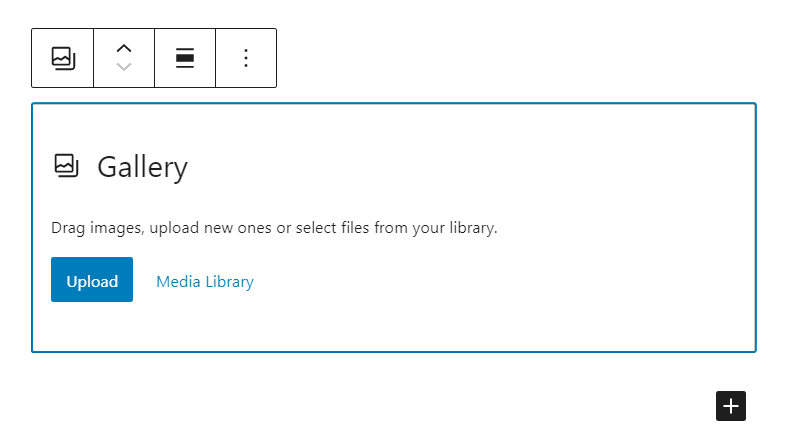The image depicts a gallery interface, predominantly featuring a white box with black letters spelling "GALLERY." At the top of this box, there is an icon comprising a black box with a white interior, featuring a squiggly line and an outline resembling an 'L'. Above this icon, there's an upper circle, an upper arrow, and a lower arrow. 

On the right-hand side of the box, a thick black rectangular button is present with lighter markings — a straight black line on both the top and bottom edges, and three dots contained within another box. Inside the main gallery area, there are instructions to "drag images, upload new ones, or select files from your library." 

An actionable upload button, colored blue with white lettering, is also visible. The interface features a blue-highlighted "Media Library" option that appears to be clickable for accessing more information. Below this main gallery box, on the right side, there is a small black box containing a white plus sign.